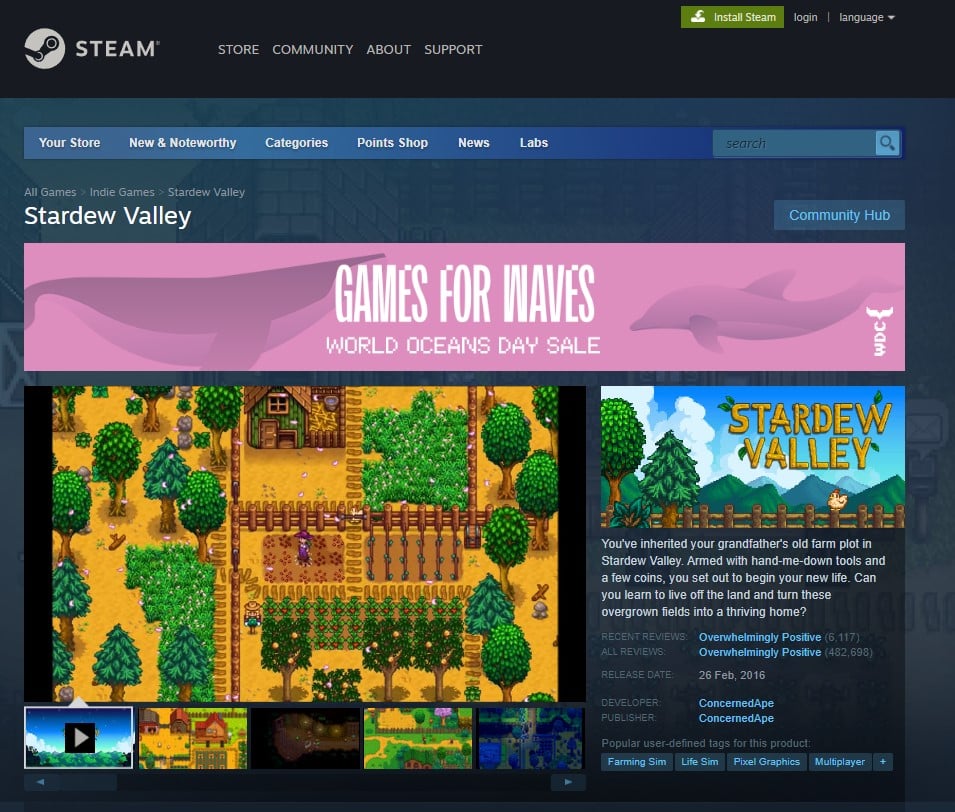The image displays a webpage of the Steam platform, with a dark blue background. At the top, a banner spans from the left to the right edge of the screen, bearing the Steam logo and name in the top-left corner. Adjacent to the name, four main categories are listed in white font: Store, Community, About, and Support. On the right side of the banner, a green button labeled "Install Steam" in white font is prominently displayed. Directly beside it, options to log in and switch the language are visible, also in white font on the black background.

Directly below, a thin blue banner contains additional categories: Your Store, Noteworthy Categories, Points Shop, News, Labs, and a search box. The page shown is dedicated to the game "Stardew Valley". An advertisement for the "Games for Waves: World Oceans Day Sale" is featured prominently. On the right-hand side of the page, detailed information about "Stardew Valley" is provided, while the left side showcases various in-game screenshots, offering a glimpse into the gameplay experience.